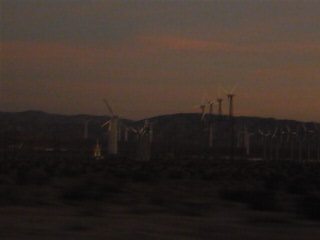In this dimly lit photograph, the dark, almost silhouette-like scenery captures a distant array of windmills scattered across a rolling hillside. The night sky above transitions from a dark gray to a faint grayish-blue and grayish-red-orange hue, implying it may be nighttime. The bases of the turbines are predominantly white, with some appearing black, creating a contrasting effect against their white blades. The windmills vary in elevation and size, some seemingly perched higher on the hill or being larger than others. The bottom left of the image shows land, possibly dirt and brush-covered, faintly appearing in the dark foreground. The overall ambiance of the photo is one of serene obscurity, with minimal light making it challenging to decipher specific details.